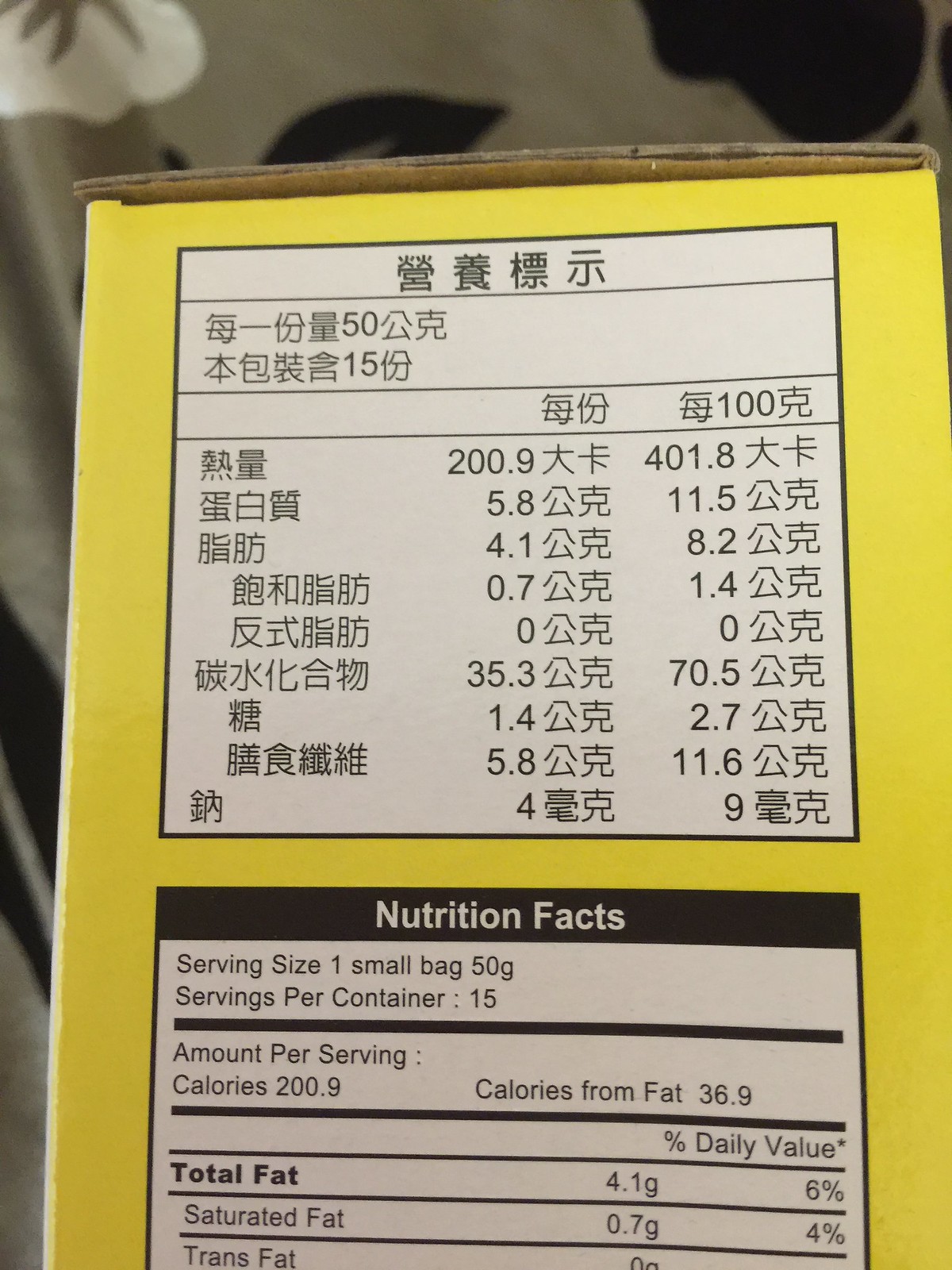The image depicts the side of a bright yellow cardboard box, featuring both Asian characters and English nutritional information. The box is cheerfully yellow and contains a prominent white section at the top with Asian lettering—likely Japanese—divided into two columns with numbers interspersed among the text. Below this is a second white box bordered with a thick black line, labeled "Nutrition Facts" in bold white letters. In black text on a white background, this section provides detailed nutritional information: serving size (one small bag, 50 grams), servings per container (15), amount per serving (calories 200.9, calories from fat 36.9), and daily values for total fat (4.1g at 6%), saturated fat (0.7g at 4%), and trans fat (0g). The upper edge of the box reveals the typical manila color of the cardboard interior. In the background, a curtain with black splotches is faintly visible.